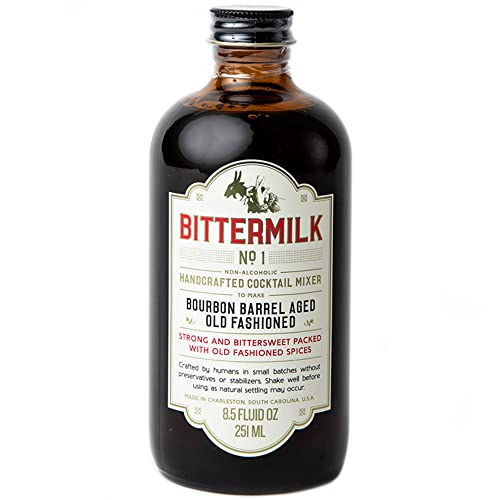The image showcases a close-up photograph of a glass bottle containing a dark brown, blackish liquid, identified as a non-alcoholic handcrafted cocktail mixer. The bottle features a silver screw-top lid and some bubbles are visible at the top. The most prominent element is a large white label with a design that includes hands making shadow donkeys. The label’s main text, "Bittermilk No. 1," stands out in red, followed by smaller descriptive text. This text details the product as a bourbon barrel-aged old-fashioned cocktail mix, characterized by its strong and bittersweet flavor and packed with old-fashioned spices. It is specified to be crafted by humans in small batches without preservatives or stabilizers. Users are advised to shake well before using, as natural settling may occur. The bottle holds 8.5 fluid ounces (251 milliliters) of liquid. The label's text varies in size and color, giving it an antiquated appearance.